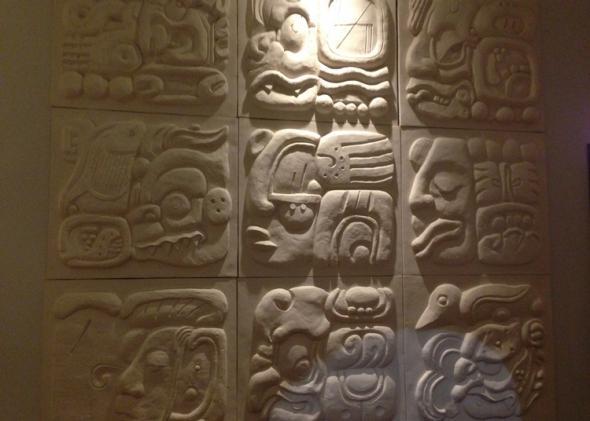This image depicts an angled view of a wall adorned with nine meticulously carved plaster tiles arranged in a 3x3 grid. Each tile features a unique, abstract design of stylized human faces, animals, and geometric shapes, reminiscent of ancient Mayan or Aztec art. The faces are characterized by pronounced features like defined noses, large lips, and closed eyes, while some tiles display birds with discernible beaks and intricate wings, as well as decorative elements like swirls, circles, and possible floral patterns.

The tiles possess a muted palette of grayish-brown, tan, and light green hues, with a notable illumination provided by a single light source positioned above the middle row. This creates a stark contrast, highlighting the central tile and casting shadows along the darker periphery of the image. The wall itself appears to be part of a plain, possibly white concrete structure, suggesting this could be an exhibit within a museum, dedicating modern lighting to emphasize the archaeological aesthetic of the artwork. A subtle, white transparent semicircular shadow in the bottom right corner of the image hints at light reflection, adding depth to the photograph and accentuating the intricate, hieroglyphic-like carvings.